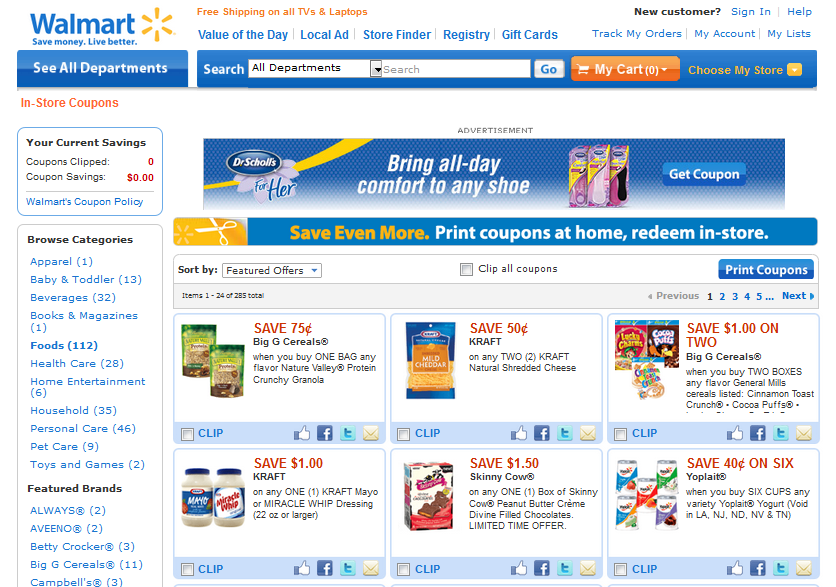The image is a Walmart advertisement displaying the recognizable Walmart logo with the blue text and the yellow spark emblem. The headline prominently announces "Free shipping on all TVs and laptops" in bold yellow letters. Below this, blue text lists various options and links, including "Value of the Day," "Local Ad," "Store Finder," "Registry," "Gift Cards," "Track My Order," "My Account," and "My List."

Above these options, the top banner features links for "New Customer Sign In or Help." On the right-hand side, icons and prompts for "My Cart (0)," "Your Current Savings," "Coupons Clipped (0)," and "Coupon Savings ($0)" are displayed. There's also a search bar labeled "Search for all departments."

The "Browse Categories" section lists the following departments with their corresponding item counts: 
- Apparel (1) 
- Baby and Toddler (13) 
- Beverages (32) 
- Books and Magazines (1) 
- Food (112) 
- Healthcare (28) 
- Home Entertainment (6) 
- Household (35) 
- Personal Care (46) 
- Pet Care (9) 
- Toys and Games (2)

Additionally, there is a breakdown of specific brands and items:
- Always (2)
- Aveeno (2)
- Betty Crocker (3)
- Big G Cereal (11)
- Campbell's (3)

Highlighted promotions include:
- "Big G Cereal: Save 75%"
- "Kraft: Save 50% on any two Kraft Natural Shredded Cheeses"
- "Big G Cereal: When you buy two boxes, any flavor, you save $1"

This comprehensive display aims to inform customers of ongoing deals and facilitate a seamless online shopping experience.